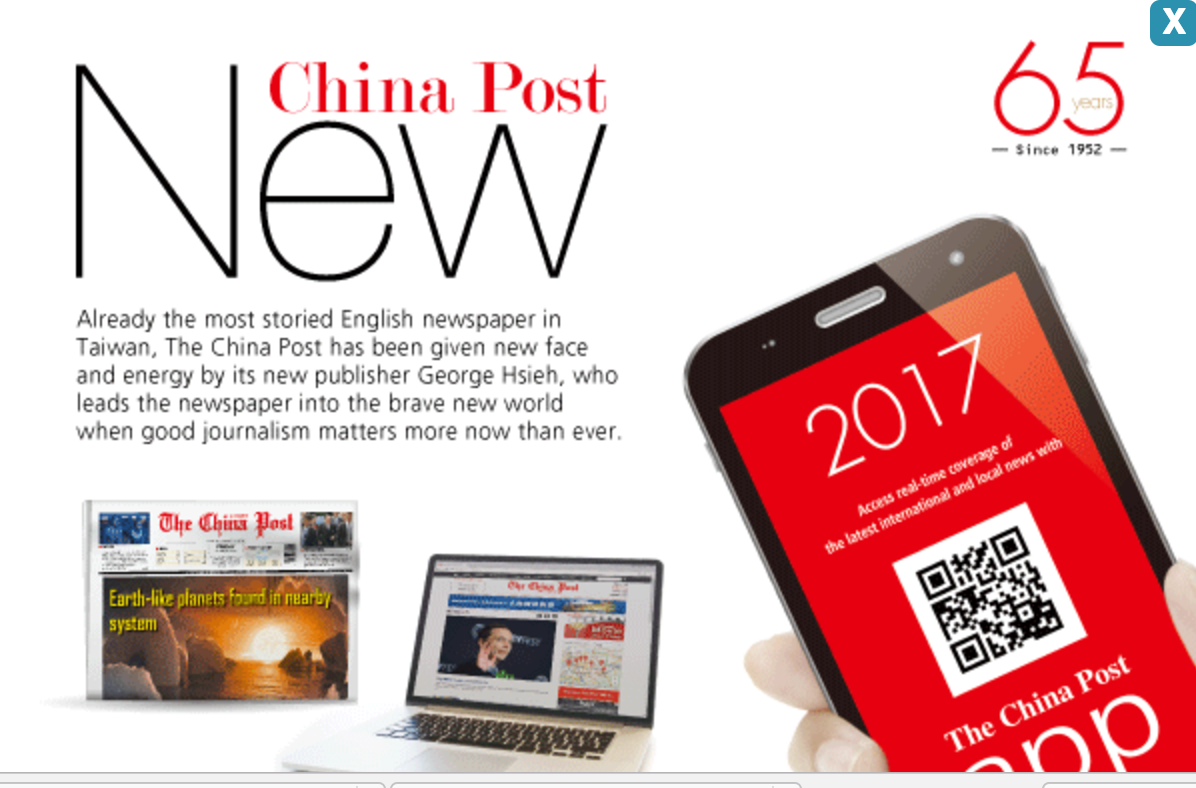The image captures the webpage of the China Post, prominently displaying the title "China Post" in red print with capitalized letters "C" and "P" at the top. Below this title, a large letter "N," the initial of the word "new," stands out. The accompanying text reads, "Are you the most storied English newspaper in Taiwan? The China Post has been given new face and energy by its new publisher, George Hsieh, who leads the newspaper into the brave new world when good journalism matters more now than ever."

Below this section, an image of the newspaper with the title "The China Post" can be seen alongside a laptop showing the same webpage. To the right, a small blue square with a white "X" and the text "65 years, since 1952" is visible. Additionally, there is an image of a hand holding a cell phone against a red background displaying the year "2017," a QR code, and the phrase "The China Post app" in white text.